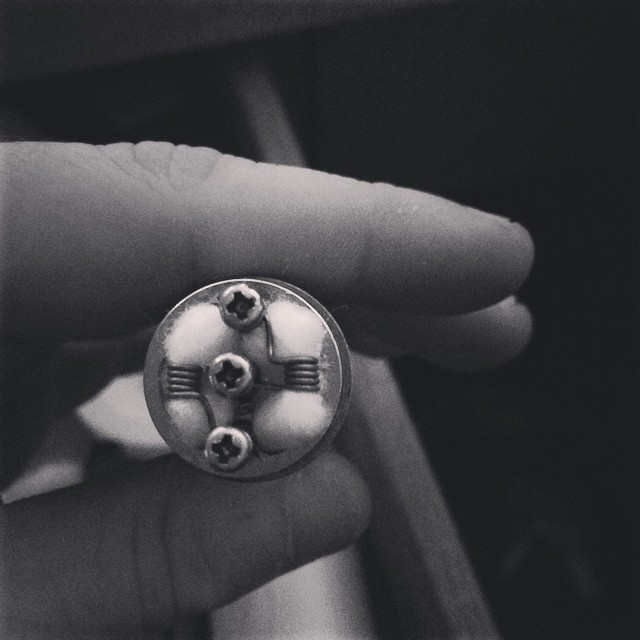The black and white, grainy image depicts a close-up detail of a tiny, round metal object, held delicately between a person's thumb and index finger, which appear from the left side of the frame. The object, which is nestled tightly within the grasp of the fingers, appears to be some form of screw assembly or possibly a nail with components attached. It is circular in shape with three screws aligned vertically from top to bottom in the center of the object, each bearing a Phillips screw head. On either side of these screws are springs, and there is a fluff-like material, potentially cotton, interspersed with the metal parts. The scene is in grayscale, presenting a spectrum of light to dark gray tones and lacking color. The background is black, adding contrast and emphasizing the miniature size of the object. The context and exact identity of the object remain ambiguous.